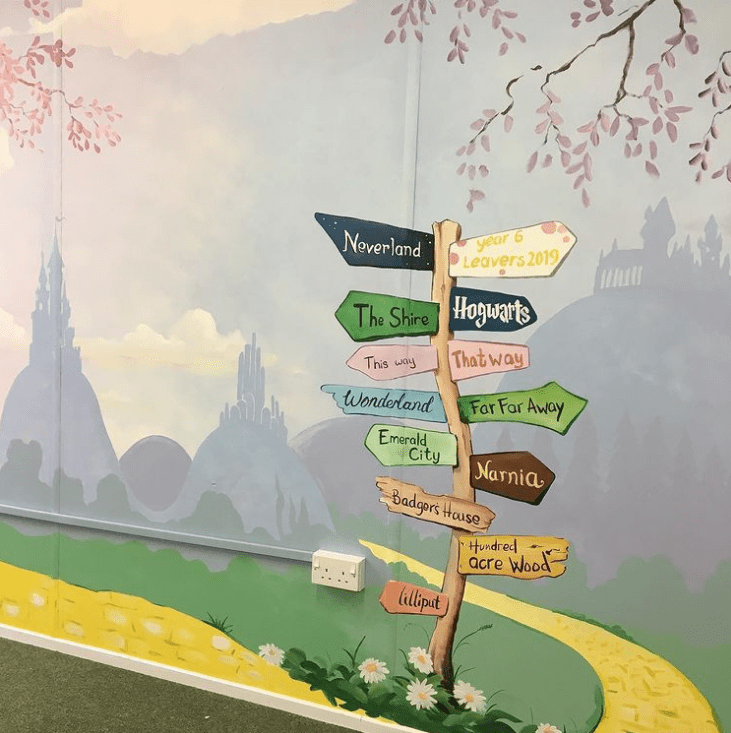The image depicts a fantastical scene with a golden path, possibly inspired by the Yellow Brick Road, leading towards a distant city adorned with three towering castles that soar into the sky. This cityscape, set amid lush greenery, trees, and mountainous terrain, evokes a sense of whimsy and adventure. Prominently featured in the foreground is a curved wooden signpost adorned with vividly colored arrows pointing in various directions. These arrows, each inscribed in distinct fonts reflective of their respective fantasy worlds, list destinations such as Neverland, the Shire, Wonderland, Emerald City, Badger's House, and Lilliput pointing to the left. To the right, the signs indicate Year 6 Leavers 2019, Hogwarts, Far Far Away, Narnia, and 100 Acre Wood, with some pointing slightly behind or off to the sides. At the base of the signpost, white daisies add a touch of natural beauty. The whole scene is rendered in a watercolory style that emphasizes its dreamlike quality, making it appear as though it were a painting on someone's wall, complete with a visible outlet and a carpet in the lower-left corner of the image.